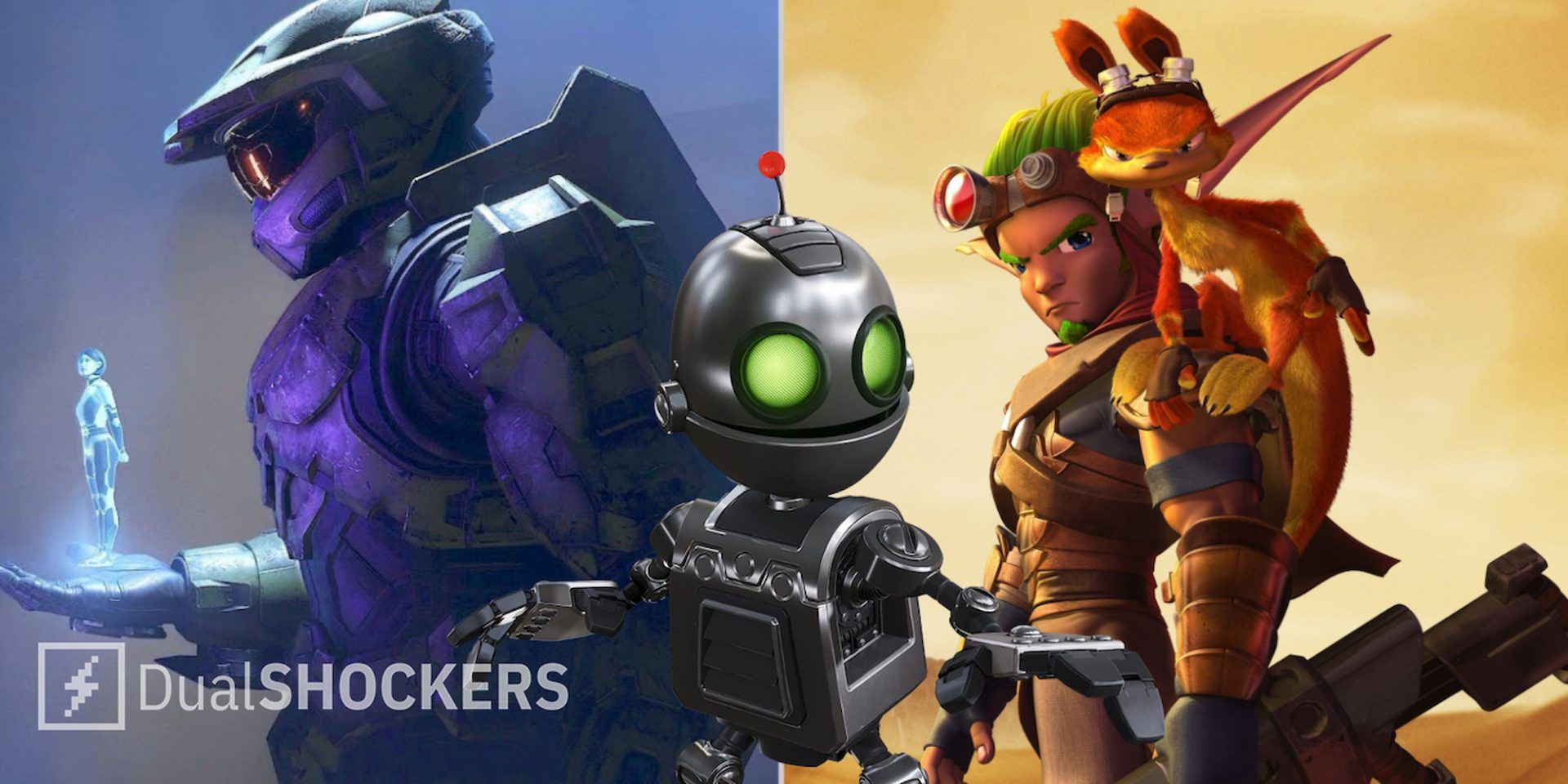The image is a computer-generated collage featuring characters from the video game "Ratchet and Clank," possibly intended as an advertisement. The collage is divided into three main sections. On the left, there is a purple-armored spaceman, viewed in profile, extending his gloved hand to project a hologram of a woman. In the center, the small robot character with a round head, green glowing eyes, and metal claw-like arms is identified as Clank, the hero's companion. The right side features Ratchet, described as an elfin spaceman in desert-brown attire, resembling a young boy with green hair. An intriguing mythical creature, resembling a space dragon or winged fox, perches on Ratchet's shoulder. The background of this section depicts a desert landscape with tan sand, adding to the sci-fi atmosphere. The image is associated with the video game and includes the text "Dual Shockers" at the bottom left.